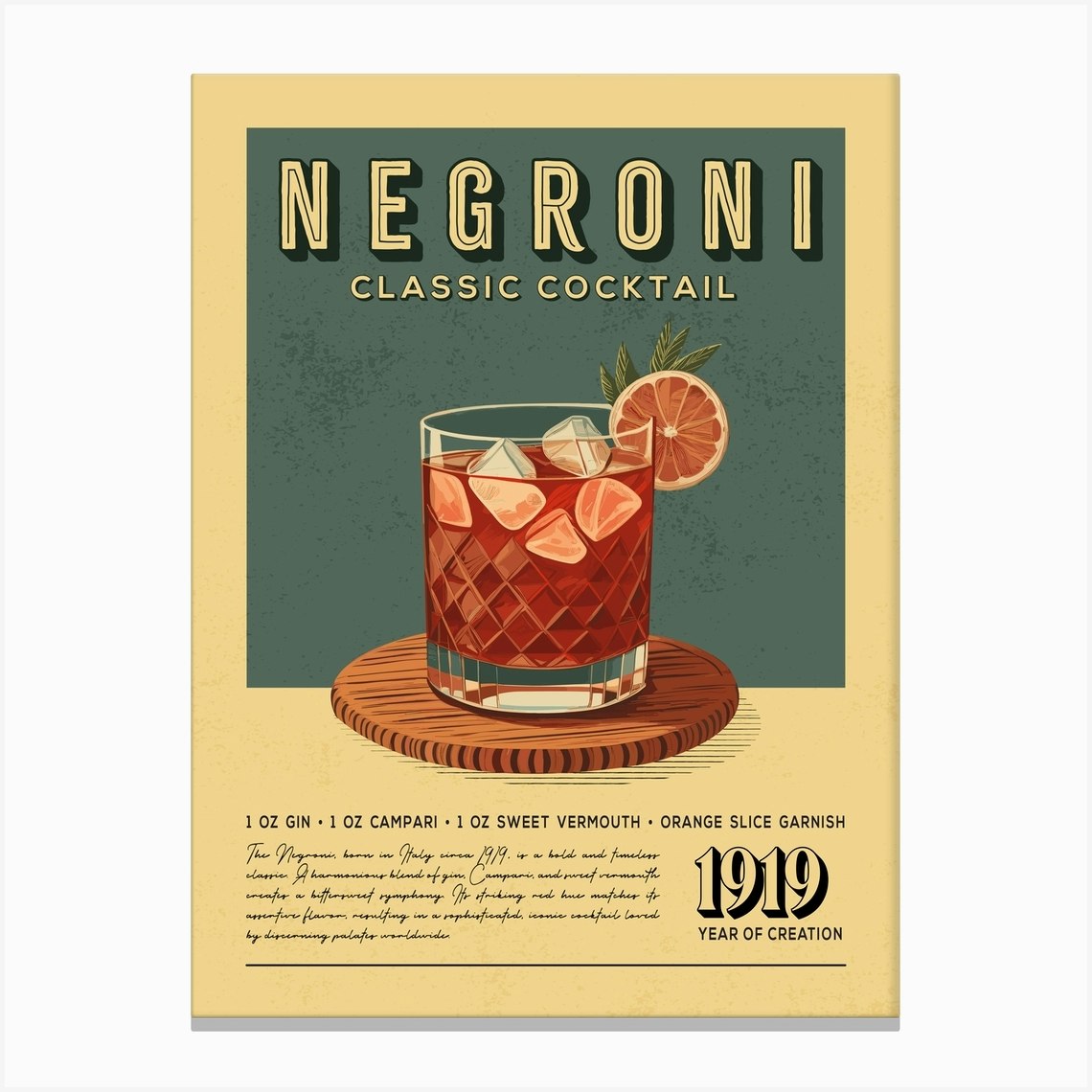The image features a vintage-style promotional illustration with a focus on the Negroni, a classic cocktail. Centered at the top in bold, cream-colored text with a black drop shadow, is the word "Negroni." Just below, in smaller cream-colored text, are the words "classic cocktail." The illustration showcases a short cocktail glass adorned with diamond shapes, filled with a brick-colored liquid, representing the one-ounce each of gin, Campari, and sweet vermouth that make up the drink. The glass holds five ice cubes and is garnished with a slice of orange with a sprig of greenery peeking behind it. It rests on a round wooden coaster which slightly protrudes from the textured, dark teal background. Underneath, in black text, the recipe is listed: "one ounce gin, one ounce Campari, one ounce sweet vermouth, orange slice garnish." To the bottom right, text outlined in black reads "1919," marking the year of the cocktail's creation. The entire scene is set against a light gray background, providing a vintage and elegant aesthetic that resembles an old newspaper or magazine clipping.